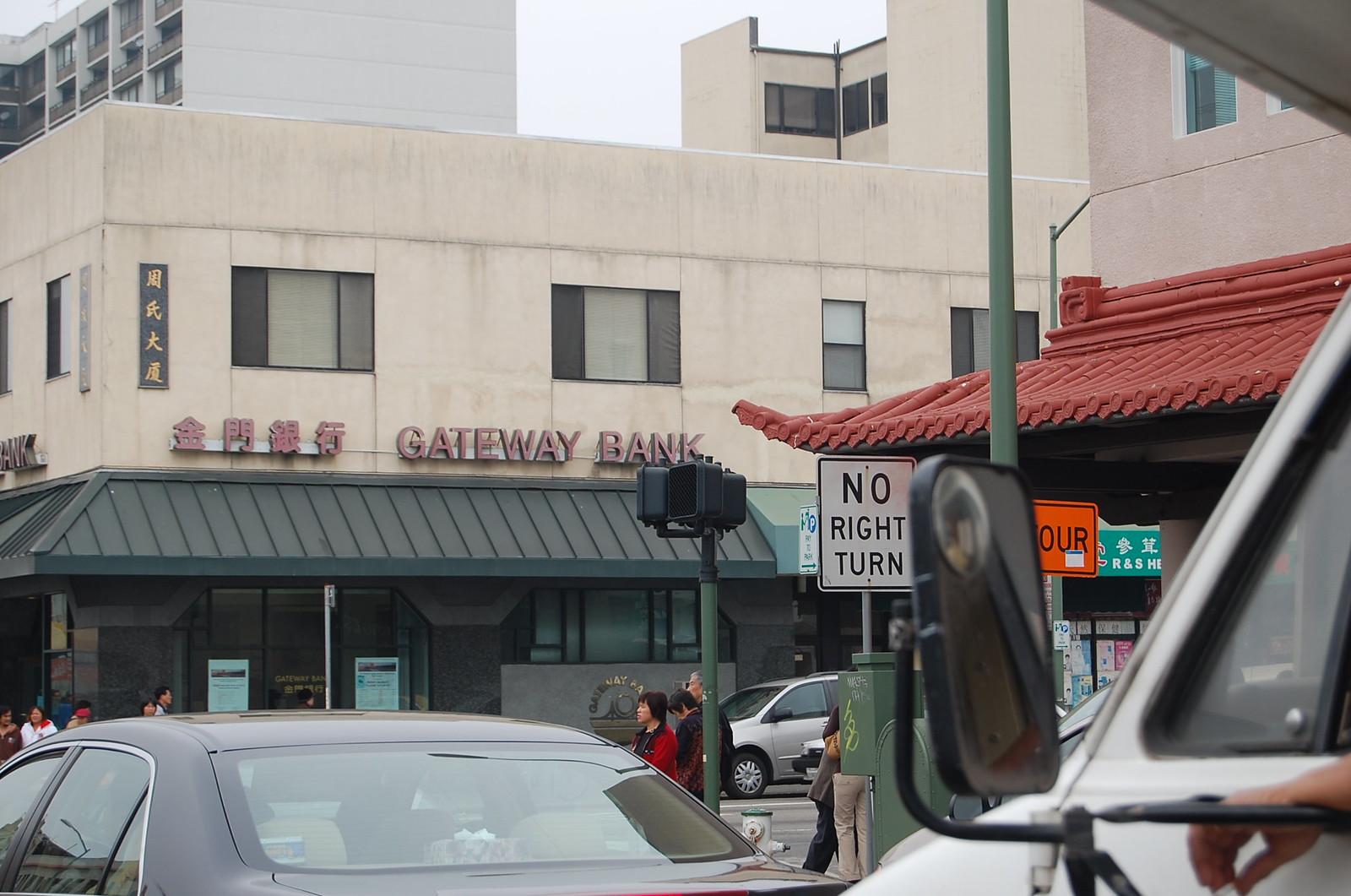The image captures a vibrant city street scene dominated by a beige building adorned with red Chinese writing and a prominent "Gateway Bank" sign on the second story. The building features a green awning that overhangs its lower level, which is distinguished by windows interspersed with black marble accents extending up to the awning. In front of this building, the street is bustling with various people crossing roads and going about their day. A black car occupies the lower part of the image, partially obscuring the view of the street, while a white pickup truck can be seen behind it. Road signs are also visible, including a white "No Right Turn" sign prominently displayed. To the left, a large white building looms in the background, adding to the city's layered architectural landscape. The sky is gray, indicative of a typical overcast day, lending a bright but diffuse light to the scene.